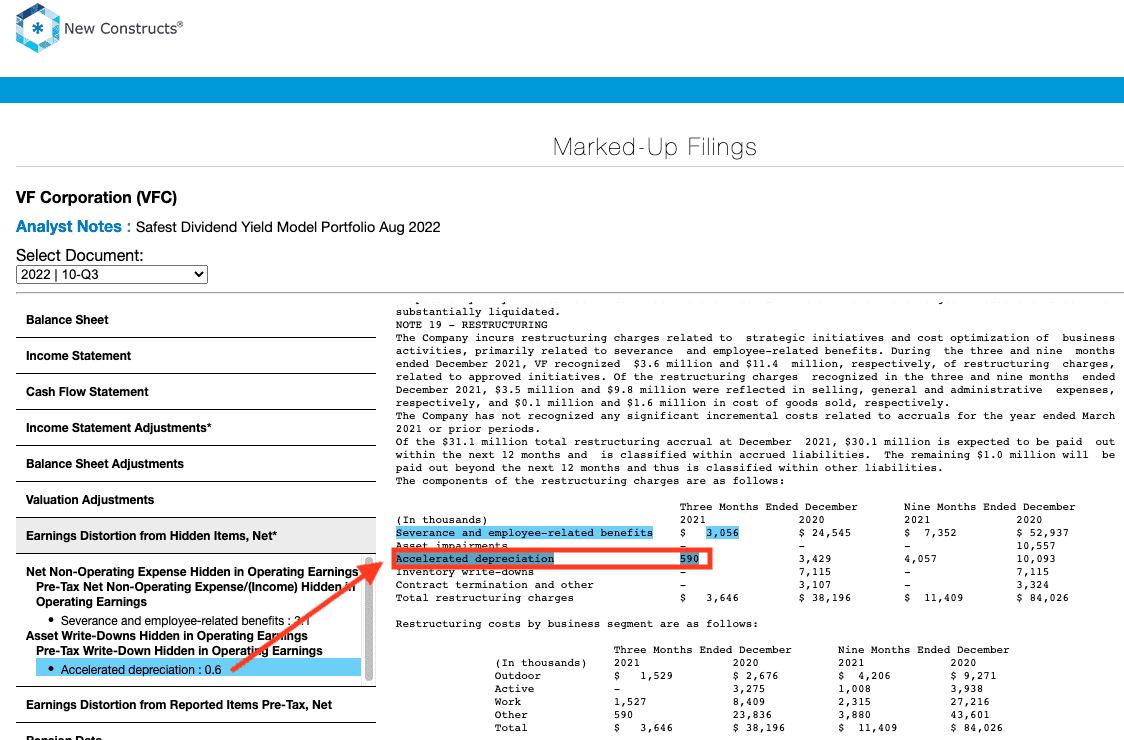The image displays a detailed financial document from VF Corporation, providing insight into their third-quarter performance for 2022. The left-hand menu includes categories such as "VF Corporation VSC," "Analyst Notes," "Safest Dividend Yield Model," and "Portfolio August 2022." A specific document dated October 23, 2022, is currently selected, marking the end of the third quarter. 

Key sections present on the document include a balance sheet, income statement, cash flow statement, and various adjustment details such as balance adjustments, valuation adjustments, and earnings distortion from hidden items. Notably, items like net non-operating expenses, pre-tax write-downs, and accelerated depreciation are highlighted for emphasis. 

The right side of the page prominently features a highlighted text pertaining to "accelerated depreciation," accentuated by a large red arrow. This section represents financial data for three-month and nine-month periods ending in September, detailing millions of dollars in transactions represented in thousands for clarity. 

The focus of this document is to shed light on accelerated depreciation, showcasing VF Corporation's substantial financial activities and adjustments within the indicated periods.